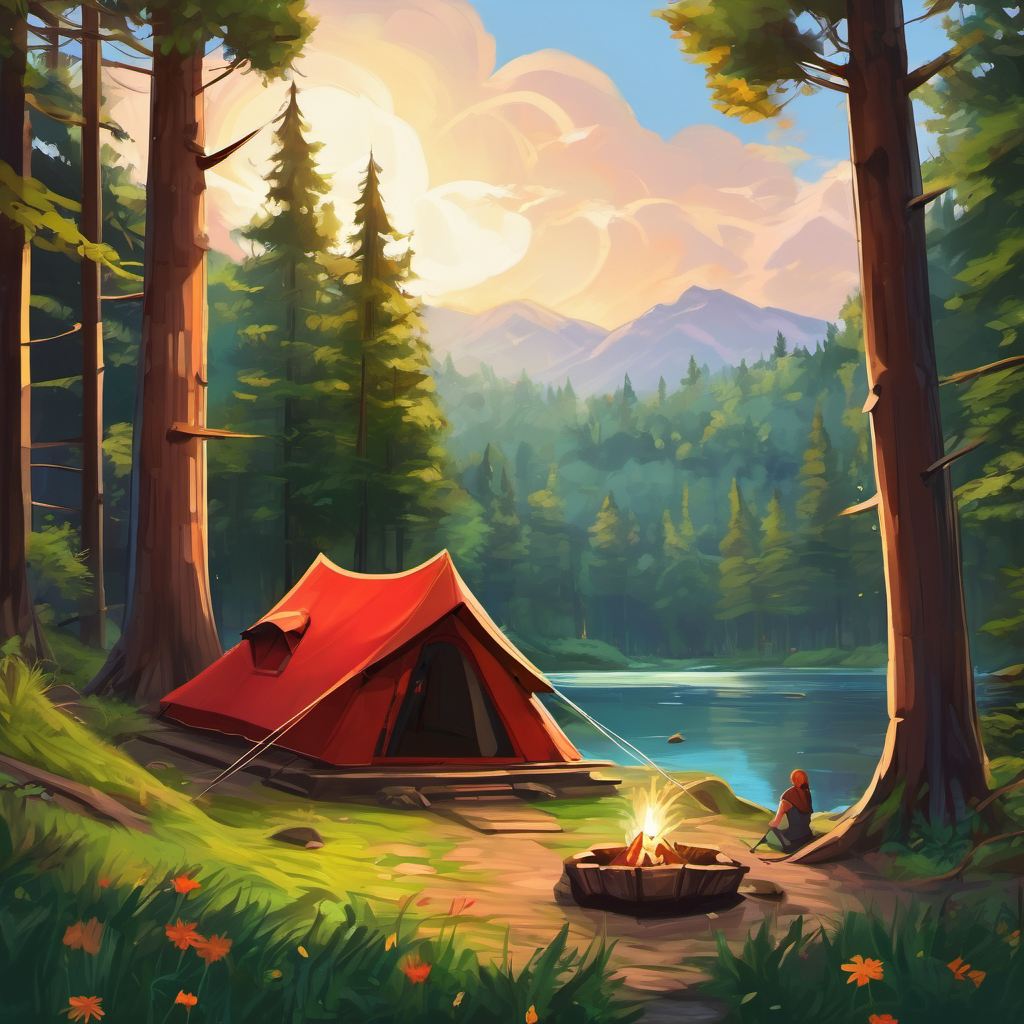This vibrant cartoon illustration depicts a serene camping scene set in a heavily forested area under a partly cloudy sky with hints of blue. Dominating the center is a large, red and slightly orange tent with a rainfly and visible internal structure, staked securely with ropes. To the right, a person clad in a scarf sits on wooden ground, gazing contemplatively at a calm, dark blue lake. A campfire blazes nearby, providing warmth and light. Surrounding the campsite, towering giant redwood trees and lush green foliage enhance the natural beauty. Bright orange and yellow flowers sprout from the tall grass in the foreground, adding a splash of color. In the distance, gray mountains rise majestically above the forest, framed by sunlit fluffy clouds, creating a picturesque and tranquil outdoor setting.